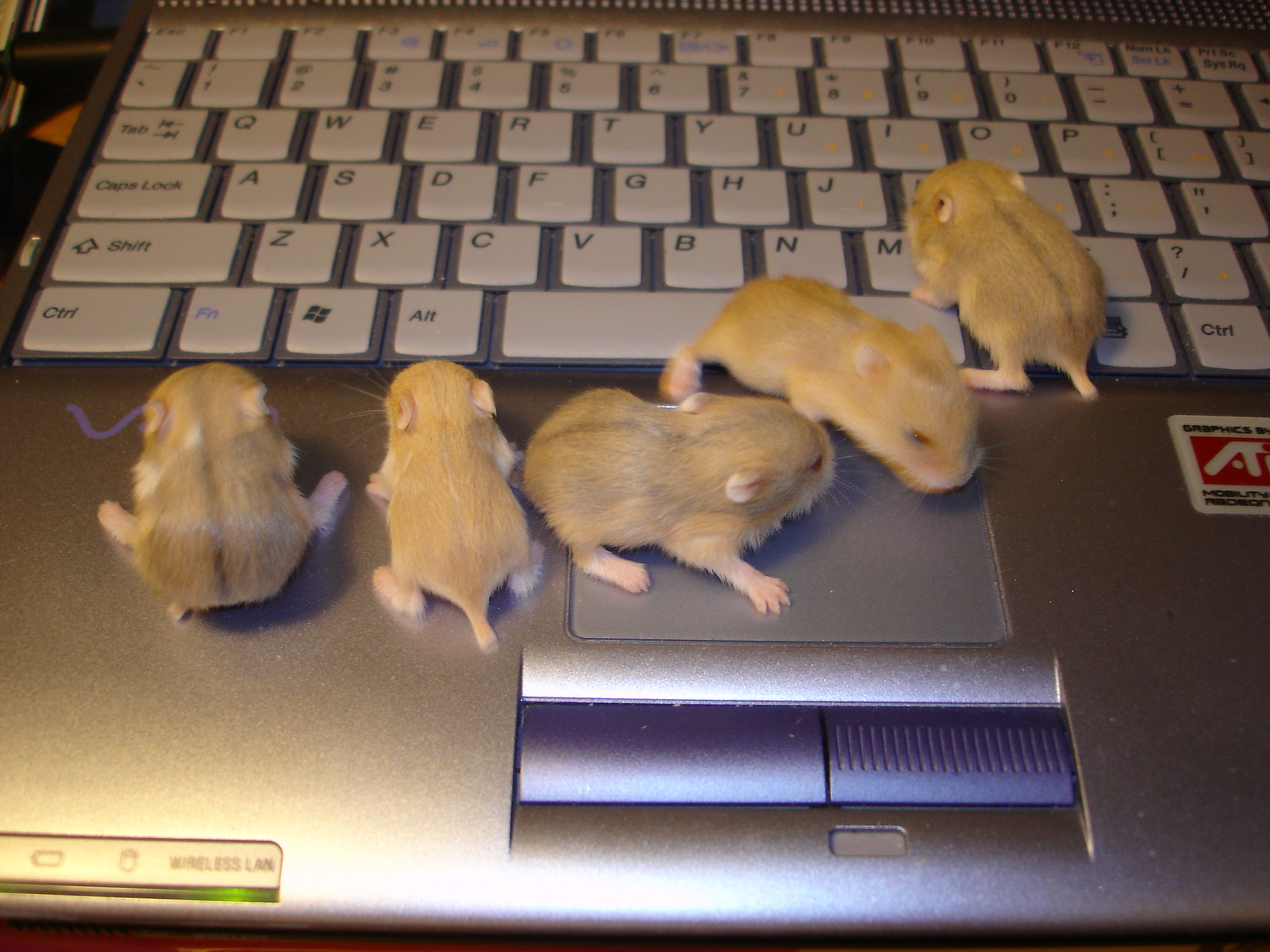The image is a detailed photograph of five small, light brown baby rodents with pink ears and paws, crawling over a silver laptop with a white keyboard. The laptop is partially cut off on the right and left edges but prominently displays its touchpad and keys. A sticker above the touchpad reads "Wireless LAN," and status lights are visible in the lower left corner. The rodents, which might be either baby mice, hamsters, or chipmunks, have very short tails and some have a faint black stripe down their backs. Their exact species is unclear, but they appear very young and are distributed across the device: one on the keyboard near the spacebar, two on the touchpad, and the others on the laptop surface around the touchpad. The scene appears chaotic yet endearing, capturing the rodents' curious exploration of the laptop.